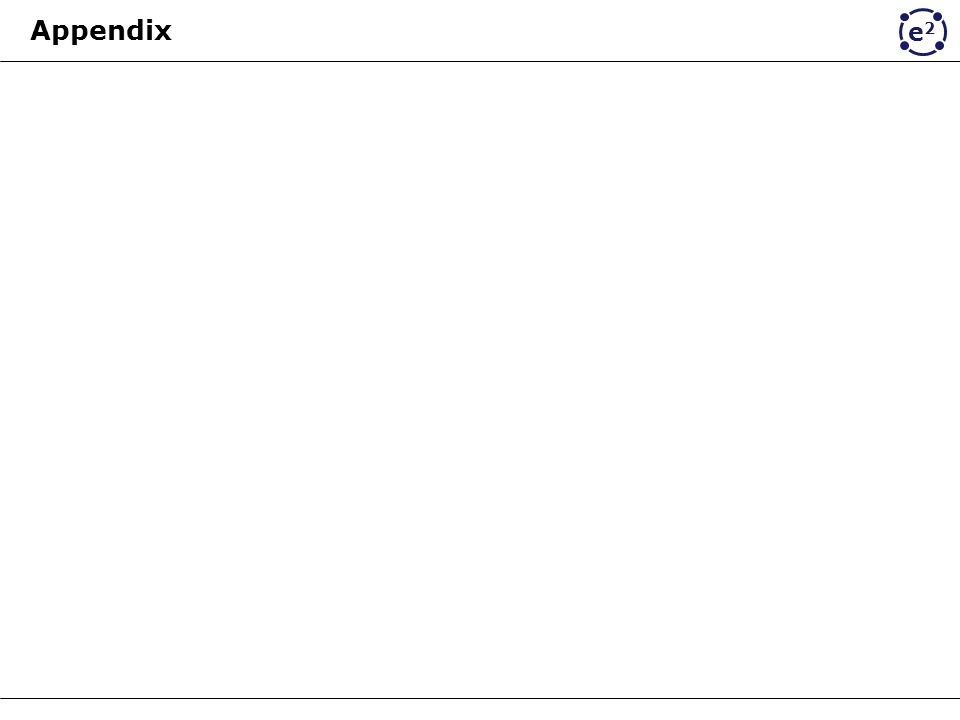This image appears to be a screenshot, likely from a webpage or a smartphone display. At the top, there is a clear, prominent header that reads "Appendix" in black print against a white background, with the 'A' capitalized and the rest of the letters in lowercase. Below this header, a horizontal gray line extends seamlessly from the left edge of the image to the right.

In the upper-right corner of the image, a small, navy blue lowercase 'e' is visible, which is accompanied by a superscript '2', indicating "e squared". Surrounding this element is a circle marked by four evenly spaced blue dots along its perimeter.

The bottom of the image features another horizontal gray line, identical in thickness and style to the one near the top. The central section of the image between these two lines is completely blank, creating a stark contrast with the detailed elements above and below it.